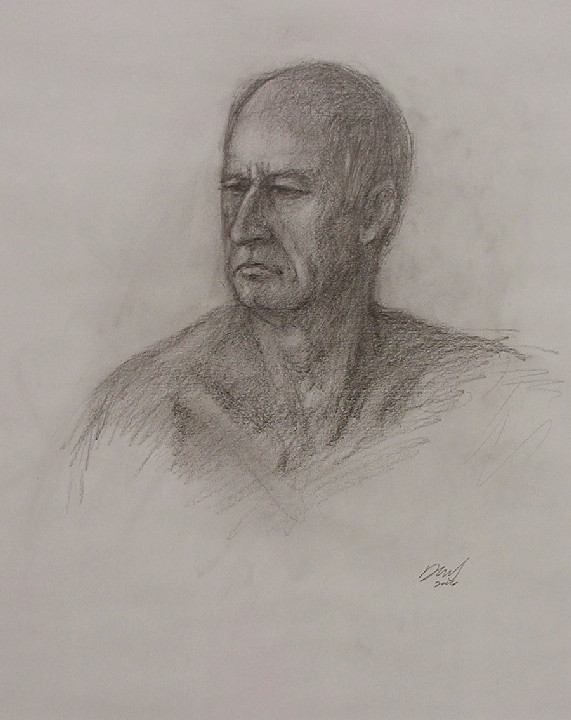The image is a hand-drawn, grey pencil illustration of a man, captured in a portrait that appears to be scanned into a computer. The piece of paper fills the entire frame, featuring the head and shoulders of the male figure. The man, likely in his late middle age to older, is depicted with his face turned to the left, looking diagonally off into the distance with a rather frowning, stern expression. His lips are turned downward at the sides, giving him a sneering or disgusted look. The figure has thinning hair or appears bald, revealing his bone structure prominently. Both eyes, dark and open, are clearly visible along with his left ear; the right ear is obscured. Only a hint of his shoulders and the top of his chest is sketched, leaving the impression of an unfinished garment that appears toga-like. The lines and shading around the figure dissipate into rough, light pencil marks, adding texture or shadow effects. On the bottom right of the artwork, there is a stylized, italic signature that seems to read "day" or something similar, accompanied by an unclear date that might be 2006.